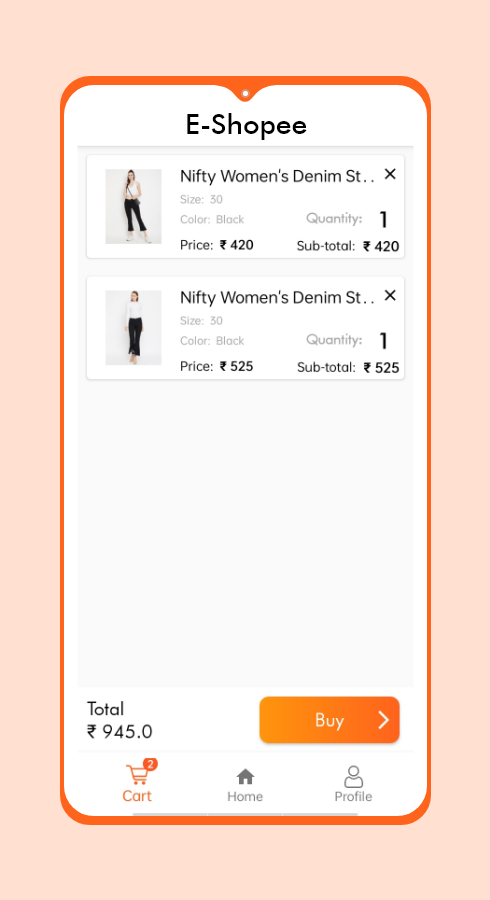This image is an advertisement for an online sales site, set against a peach-colored background. At the center of the image is a stylized drawing of a cell phone depicted in a dark orange silhouette, oriented in a portrait format. At the top, a small triangle intrudes into the white screen area, representing the camera placement.

The screen of this illustrative cell phone is white, with the site name "E-SHOPE" centrally aligned and underlined by a thin gray line. Below this header, a pale gray block contains two white segments, each featuring a thumbnail image.

The top segment displays a thumbnail of a woman dressed in dark pants and a light-colored top. Next to the thumbnail, the text reads, "Nifty Women's Denim..." with additional details such as size, color (black), quantity (one), and price (420 units of an unspecified currency), leading to a subtotal of 420.

The adjacent segment below similarly shows a woman in black pants and a white top, with the same "Nifty Women's Denim..." label. The details provided include size, color (black), quantity (one), priced at 525 units, resulting in a subtotal of 525.

Scrolling down to the bottom of the image, on the left side it reads "Total" followed by a currency symbol and the amount 945.0. On the right side is an orange gradient block transitioning from light to dark orange horizontally. Inside this block, the word "Buy" is displayed in white, accompanied by a right-facing arrow, also in white. 

At the bottom of the screen, navigation options are visible: on the left, a cart icon indicating two items, in the center, a home symbol with the label "Home," and on the right, a profile icon represented by a person drawing, labeled "Profile."